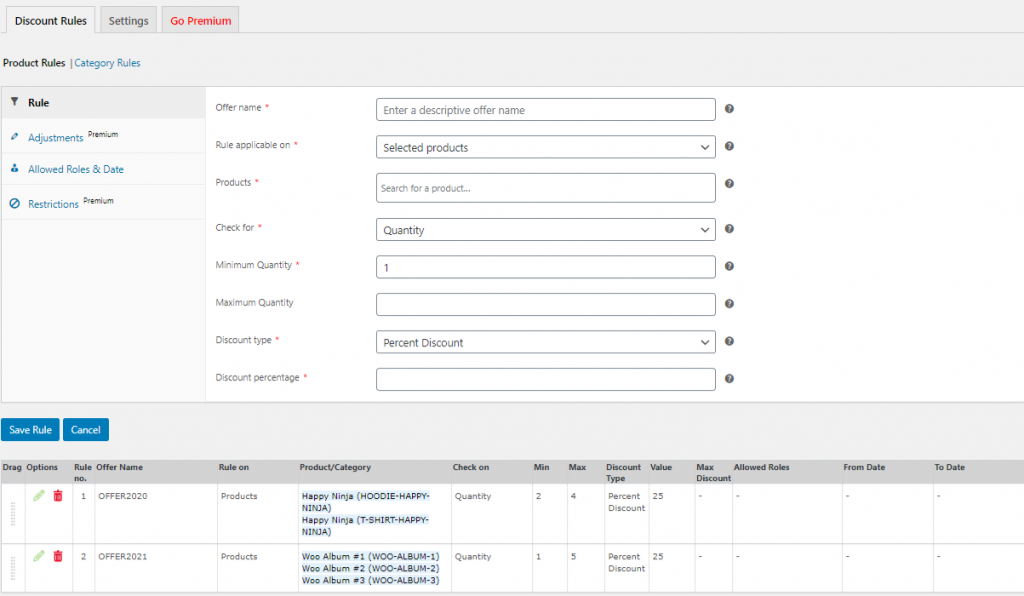The image depicts a minimalistic settings page for an e-commerce platform characterized by a clean and straightforward design with a white and light gray color scheme, accented by black text and blue buttons and links. At the top of the page, there's an option to "Go Premium."

On the left-hand side, a vertical menu lists several sections including "Discount Rules," "Settings," "Go Premium," "Product Rules," and "Category Rules." Apart from these, there are other subsections like "Rules Adjustments," "Allow Role and Date Restrictions," and "Adjustments & Restrictions," indicating these might be premium features.

The main section of the page contains multiple text fields such as "Offer Name," "Rule Application on Products," "Check for Minimum Quantity," "Maximum Quantity," "Discount Type," and "Discount Percentage." These fields are devoid of any user input, displaying only their default placeholder text. Adjacent to each field is a small question mark icon, likely to provide further explanations or guidelines when clicked. 

At the bottom of this section, there are two primary buttons: one to "Save Rule" and another to "Cancel." 

Below these buttons, the page showcases a table-like list featuring two pre-defined discount rules complete with their respective settings. This list resembles an Excel spreadsheet, including columns and rows to systematically display each rule's details and configurations. 

Overall, the page is designed to manage discount rules and product settings, offering easy access to premium features and detailed customization options.